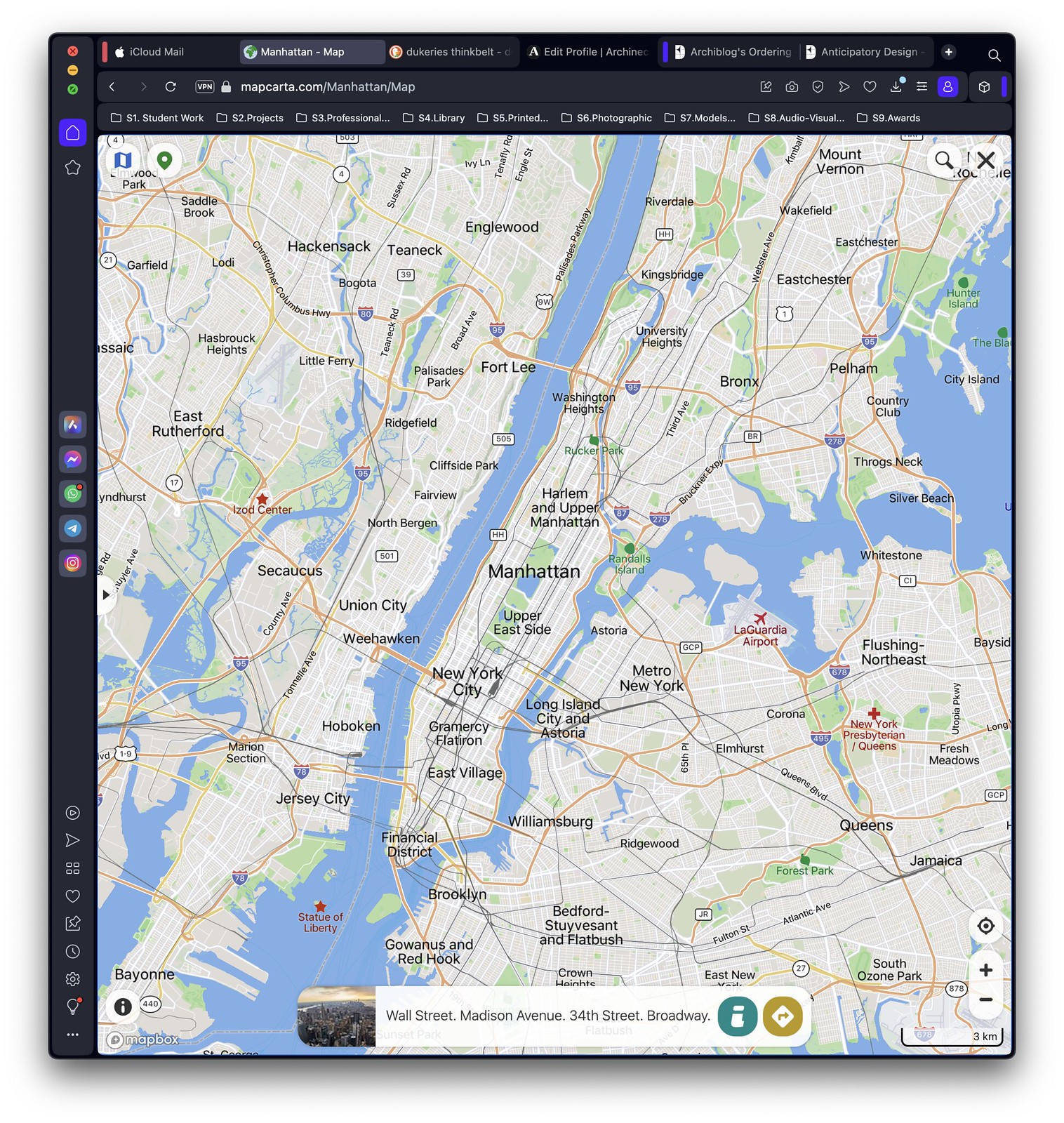This detailed map of New York prominently features Manhattan at its center. Surrounding Manhattan, the map displays the neighboring boroughs, towns, and cities, including Hackensack and East Rutherford to the west, and Flushing, Jamaica, and Queens to the east. Waterways coursing through the region are clearly delineated, alongside marked highways facilitating navigation. Notable landmarks such as the Statue of Liberty are marked with a star in the southern part of the map. To the north, the map extends to areas like Riverdale and Ernie. The map is sourced from Mapcarta.com, with the bottom section highlighting significant New York addresses including Wall Street, Madison Avenue, 34th Street, and Broadway. It is evident that the user is actively browsing for information, as indicated by the presence of several open browser tabs in the window.